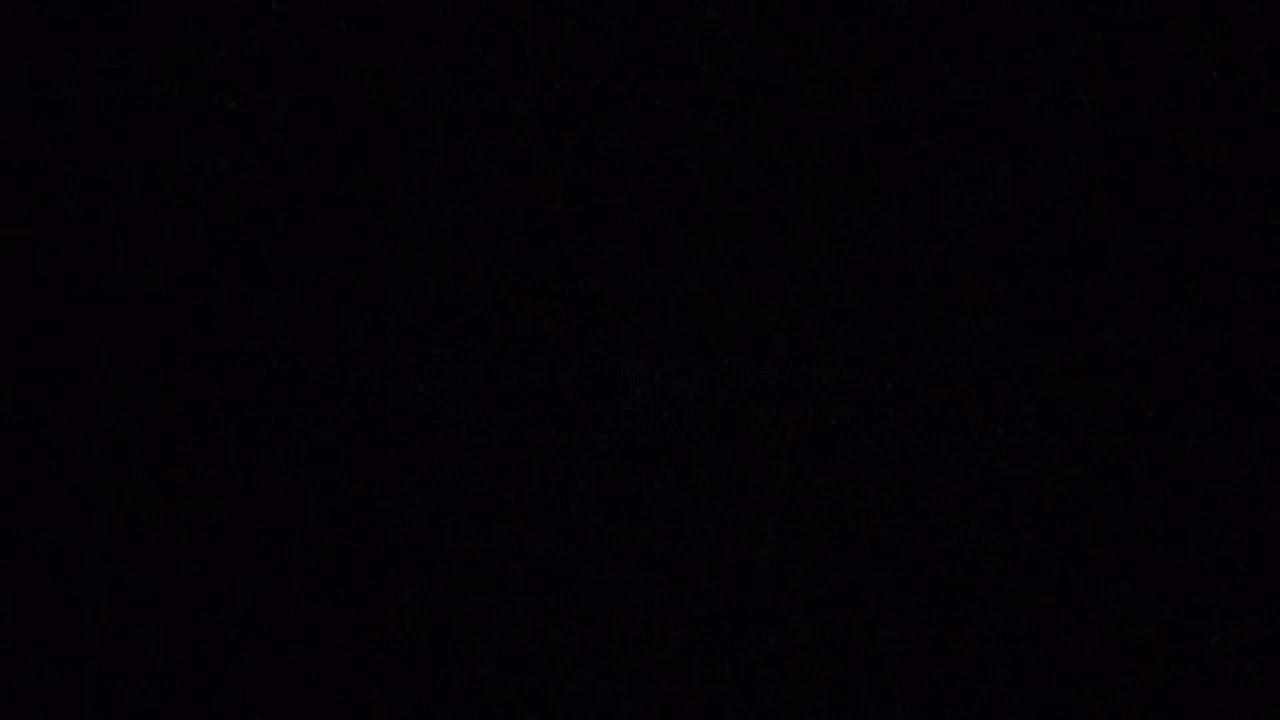The image displays a completely solid black rectangle with no discernible features, text, or objects. It is uniformly black, reminiscent of a turned-off TV screen or a chalkboard, presenting the color black in its purest form. The quality is clear and undistorted, creating a stark, unbroken expanse of darkness.